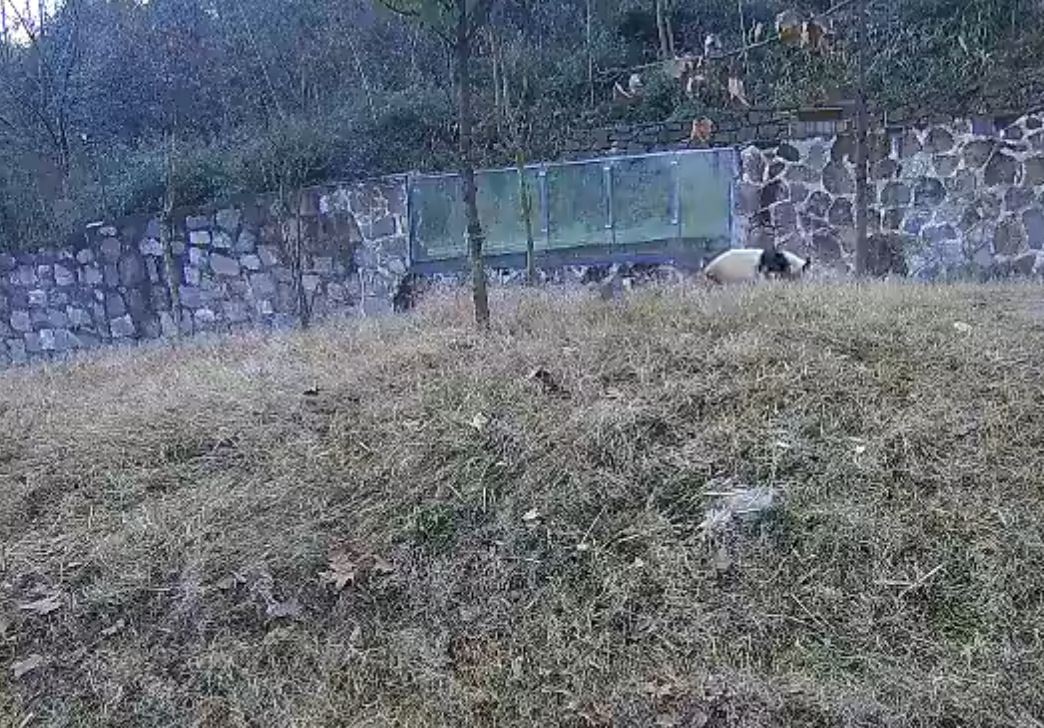The image captures a panda bear enclosure set outdoors, bordered by a meticulously crafted stone wall connected by a metal gate. The backdrop reveals a forest dense with trees, hinting at a natural, zoo-like setting. In the foreground, a grassy hill, characterized by dry and brown foliage, rises in front of the stone wall. This hill features a single, leafless tree stripped of branches. At the center near the top right, a partial view of a panda bear with its head down is visible amidst the long, dark gray and dark green grass. Scattered around the ground are small sticks, twigs, and dead leaves, adding to the enclosure's untamed look. A clear portion of the stone wall allows a few onlookers to peer inside, their presence marked by the stone terraces stepping up the rise behind them. The muted light casts a somber tone over the panda enclosure, hinting at an overcast day.